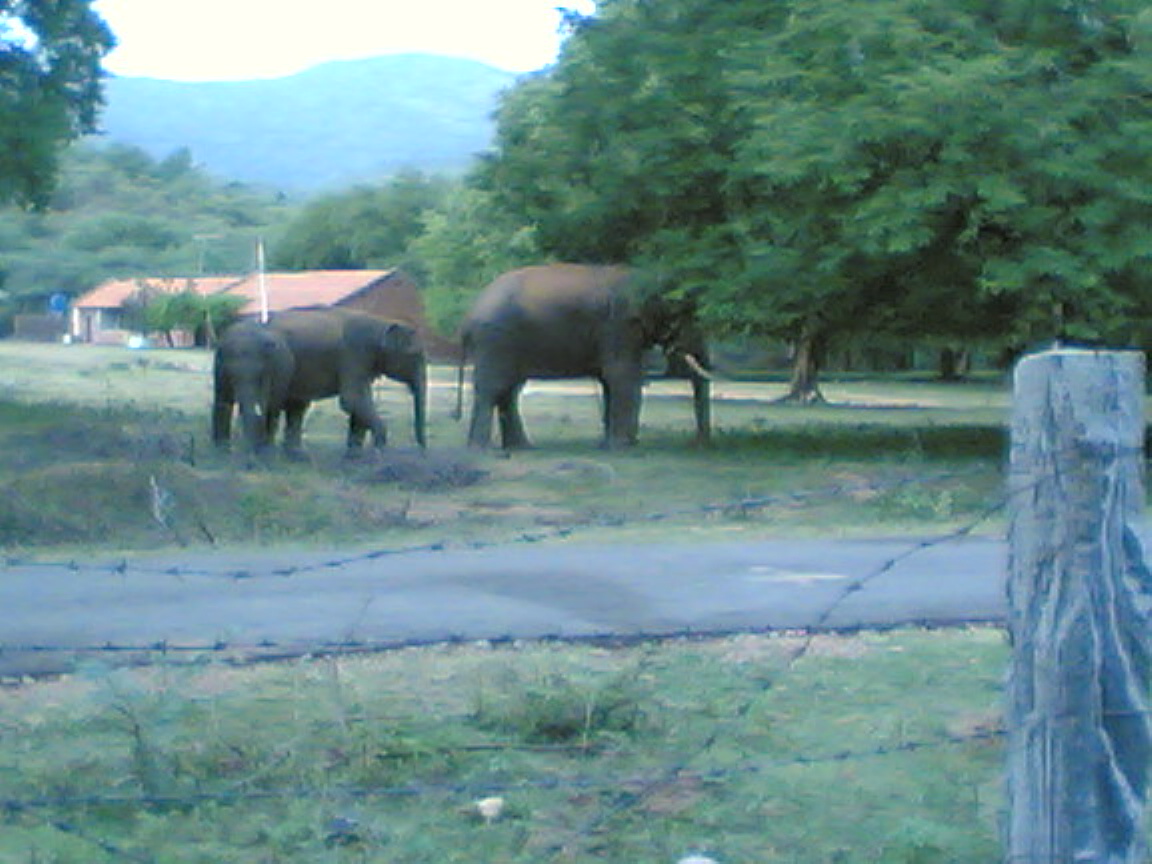In the foreground of this outdoor photograph, a wooden fence post on the right side rises halfway up the image, with a wooden slat extending horizontally to the left. Barbed wire is draped around this wooden structure, adding a rustic element. The scene transitions into a slightly overgrown grassy field, interspersed with sandy patches and dotted with what appears to be purplish wild plants. Dominating the upper right portion of the image is a grand, leafy oak tree, its overhanging branches creating a natural canopy.

The focal point of the image is two elephants in the middle of this pastoral expanse. The larger elephant, an adult with prominent beige tusks and a straight hanging trunk, stands in front, facing to the right. Slightly behind and to the left of it is a smaller elephant, likely a juvenile, following its path. The positioning and size difference suggest a familial relationship, perhaps mother and calf. Both elephants are depicted from their right side, with their flat backs and downward trunks clearly visible.

The background reveals a colorful tapestry of nature: rolling hills covered in dense vegetation, tall trees, and distant forested mountains beneath a bluish-white sky. To the left of the frame, a long, one-story building with a pitched red roof stands, likely serving as a shelter or habitation within this apparent safari park or enclosed reserve.

An asphalt road separates the grassy field from the foreground, suggesting human infrastructure within this natural setting. Overall, the image captures a harmonious blend of natural beauty and wildlife, interlaced with subtle human elements.